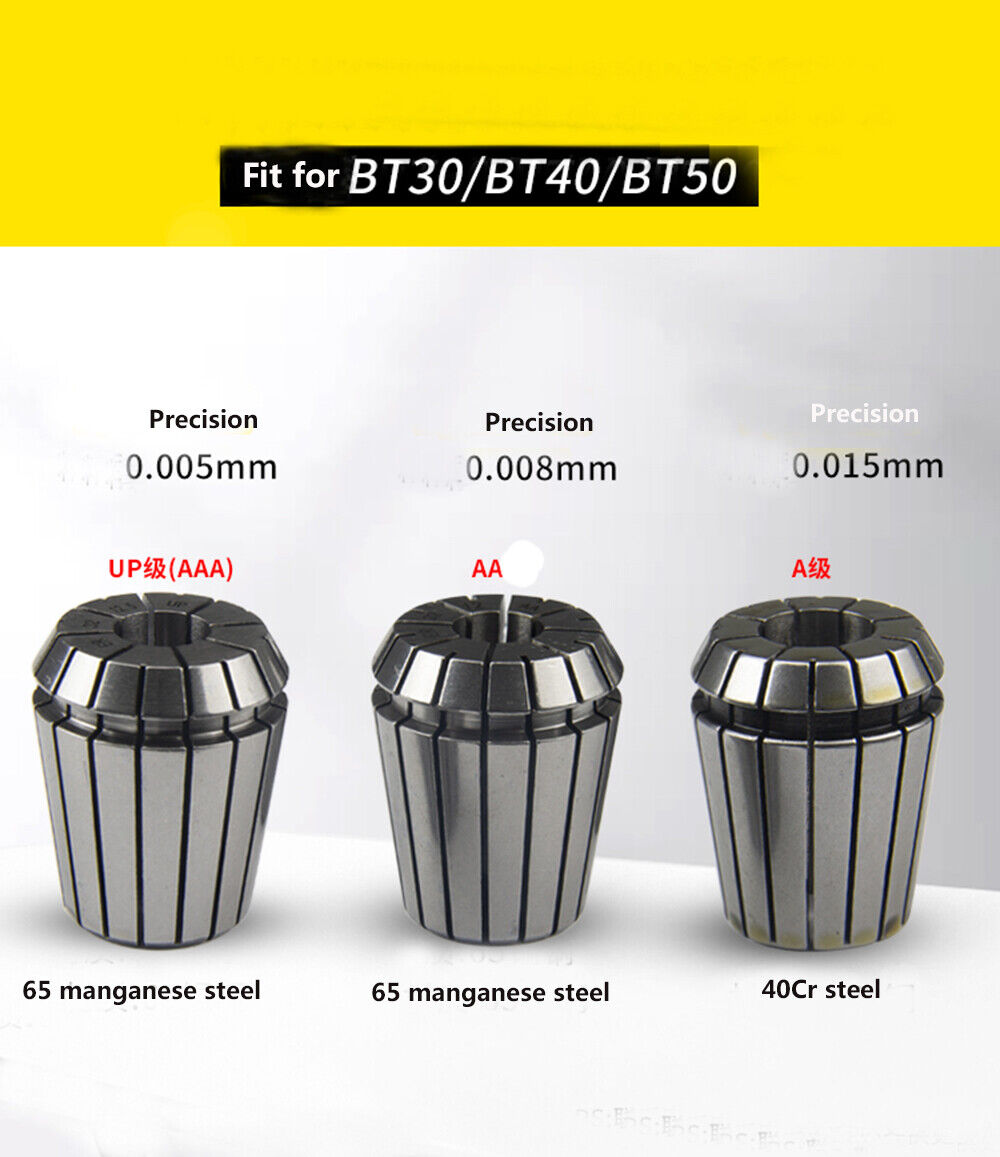The image is an advertisement, likely a digital poster, that showcases various metal tools. The ad is divided into two sections. At the top, a yellow horizontal bar stretches across the image, featuring a black bar within it with white text that reads "fit for BT30 / BT40 / BT50." Below this section, the background transitions to a grey wall and a white table on a white floor, giving a clean and professional appearance.

In the foreground, three metal cylindrical objects, which resemble vases or cans, are displayed. These objects are primarily black and grey and vary slightly in size, though the differences are subtle. Each object features the word "precision" followed by specific measurements: the first reads "precision 0.005 millimeters" and is made of "65 manganese steel"; the second reads "precision 0.008 millimeters" and is also made of "65 manganese steel"; the third object reads "precision 0.015 millimeters" but is made of "40 CR Steel." Each of these precision measurements and material details are prominently labeled above the objects. Additionally, the first and second objects share the same composition of 65 manganese steel, while the third is distinct with 40 CR Steel. 

The ad effectively highlights the precision and material quality of each tool, emphasizing the meticulous manufacturing standards. Each item appears to have unique product codes, with some featuring additional Chinese or Japanese characters, adding to the technical detail of the advertisement.